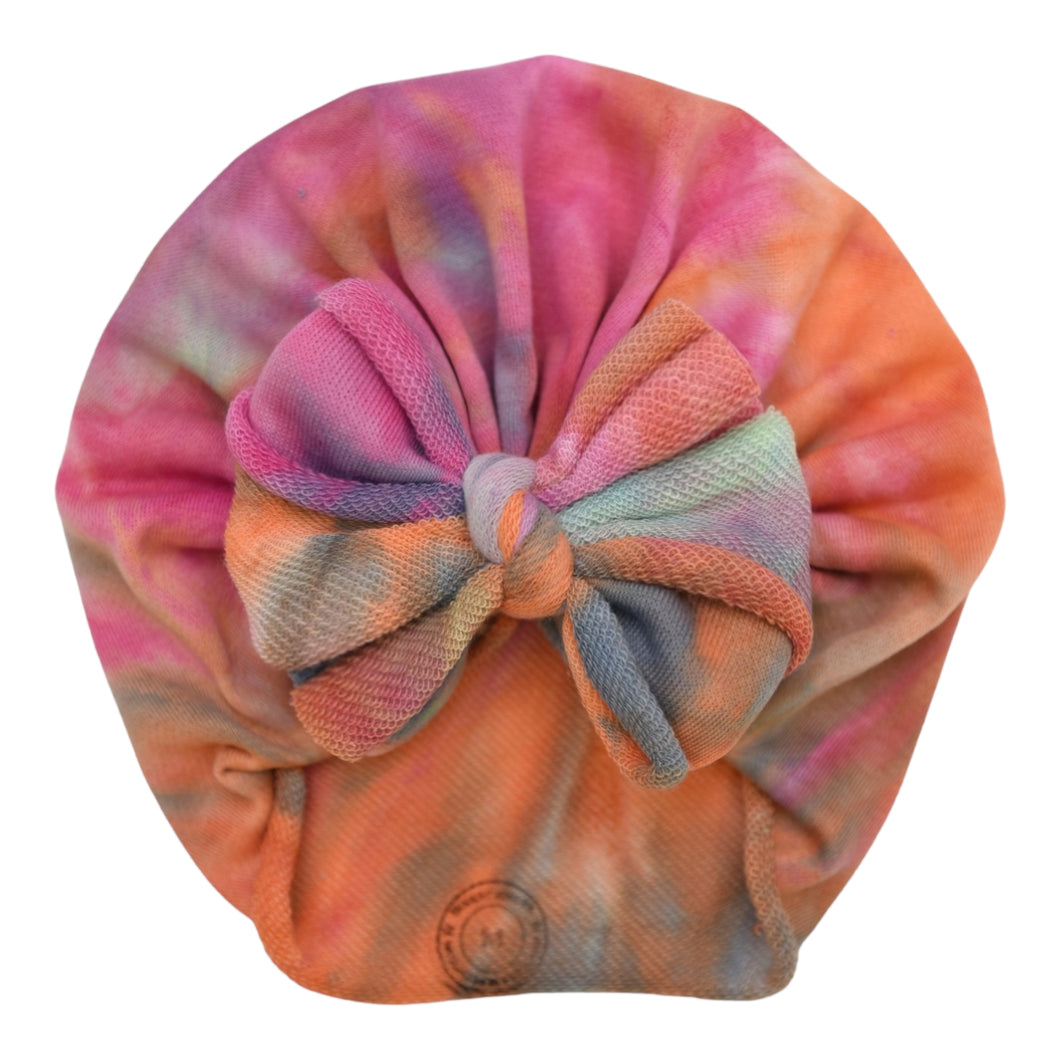This highly detailed product image showcases a vibrant, tie-dyed bonnet designed for protecting hair during sleep or from environmental elements such as wind and sun damage. Made from a soft terry cloth-like material, the bonnet features a colorful blend of orange, pink, purple, blue, green, and gray hues arranged in an eye-catching tie-dye pattern. Dominating the front of the bonnet is a large, charming bow tied from the same fabric, adding a playful and feminine touch to the headwear. The interior of the bonnet reveals a circular tag stamped with a black 'M,' indicating the medium size of the product. The background is a clean, plain white, which highlights the vivid colors and intricate design of the bonnet.